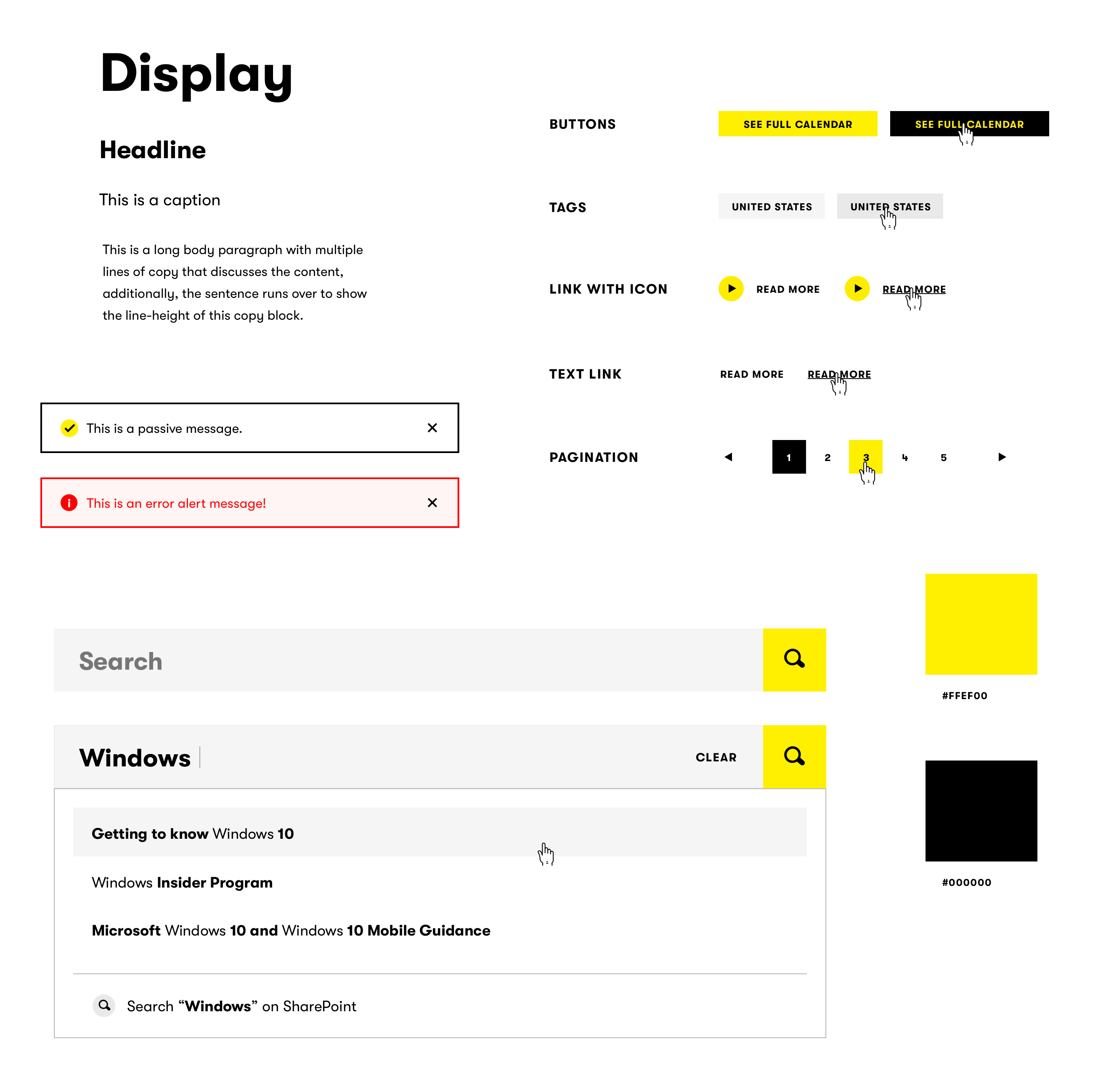The image is a vertical layout with a white background, likely illuminated by a computer screen. At the top, there is a bold block labeled "Display," followed by a slightly smaller block labeled "Headline." Below these headings is a lengthy body paragraph discussing the content, demonstrating the line height by having text run over multiple lines.

On the right side of the image, there are several bolded labels such as "Buttons," "Tags," "Link with Icon," "Text Link," and "Pagination." Under "Buttons," options include "See Full Calendar" in both yellow and black. For "Tags," there is repetition of "United States." The "Link with Icon" section features the phrase "Read More" repeated multiple times. "Pagination" shows the number "1" inside a black box and the number "3" inside a yellow box.

On the left side, there is a boxed section with the message "This is a passive message," including a yellow circle with a black checkmark. Adjacent to it, a red box contains the error message "This is an error alert message" accompanied by a red circle with an upside-down exclamation mark.

Additionally, there is a gray search bar with a yellow magnifying glass icon. Users can click "Clear" or use the search function symbolized by the yellow magnifying glass. Text associated with this search bar reads "Getting to know Windows 10, Windows Insider Program, Microsoft Windows 10 and Windows 10 Mobile Guidance," along with a note that you can search Windows on SharePoint.

On the right-hand side, there are two small squares, one yellow and one black, adding a final touch to the detailed composition of the image.